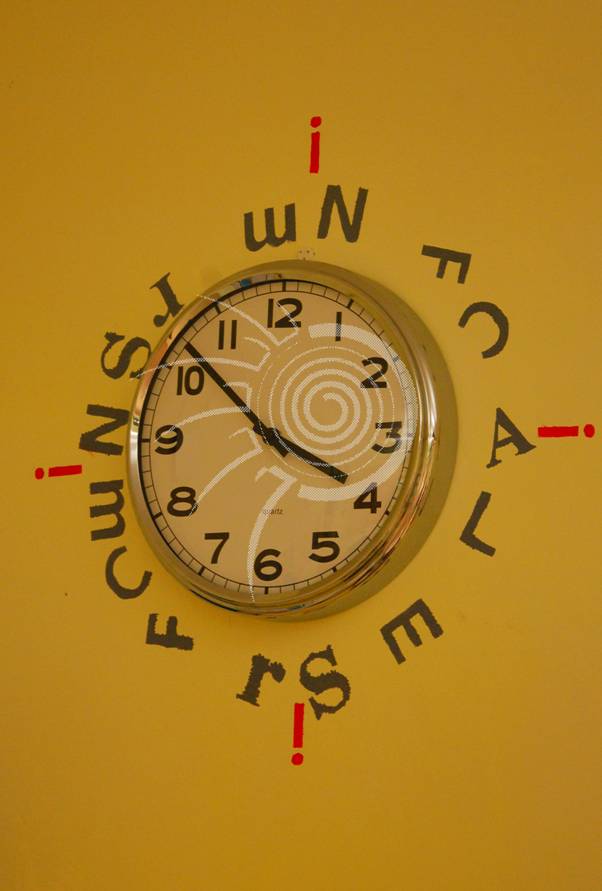This is a detailed color photograph depicting an analog clock mounted on a mustard-yellow wall. The clock itself features a very light yellow face, contrasting with its black numerals, minute hand, and hour hand. The time displayed on the clock is approximately eight minutes to four. The clock is encased in a metallic rim, adding a subtle touch of sophistication. Surrounding the clock, random letters are inscribed directly onto the wall in a circular pattern, creating an intriguing visual element. Additionally, four prominent red lines intersect the wall at the top, bottom, left, and right sides, further framing the clock and contributing to the overall composition of the image.